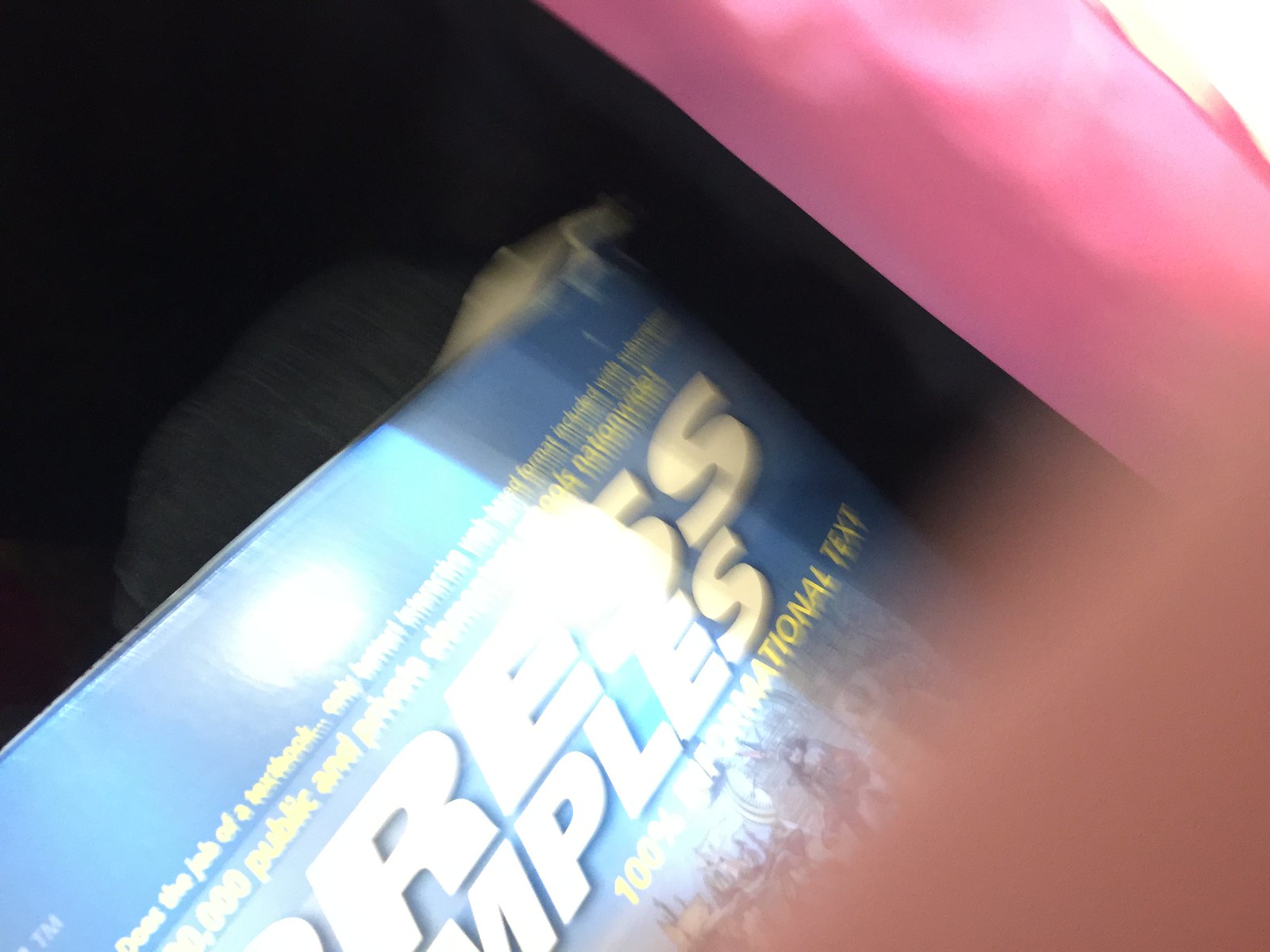The image appears slightly blurred, possibly due to motion. In the top right corner, a red object — potentially a bar or a shirt sleeve — is partially visible. On the bottom left, there's a blue box with white letters, partially legible as "R-E-S-S" and "M-P-L-E-S," suggesting the words "PRESS" and "SAMPLES." Below this, the text is unclear but might be "nutritional" or "instructional," followed by the word "text," all printed in white on a blue background. The bottom of the box features yellow letters. The background of the image is predominantly black, with the bottom right corner displaying a blurry reddish-tan hue.